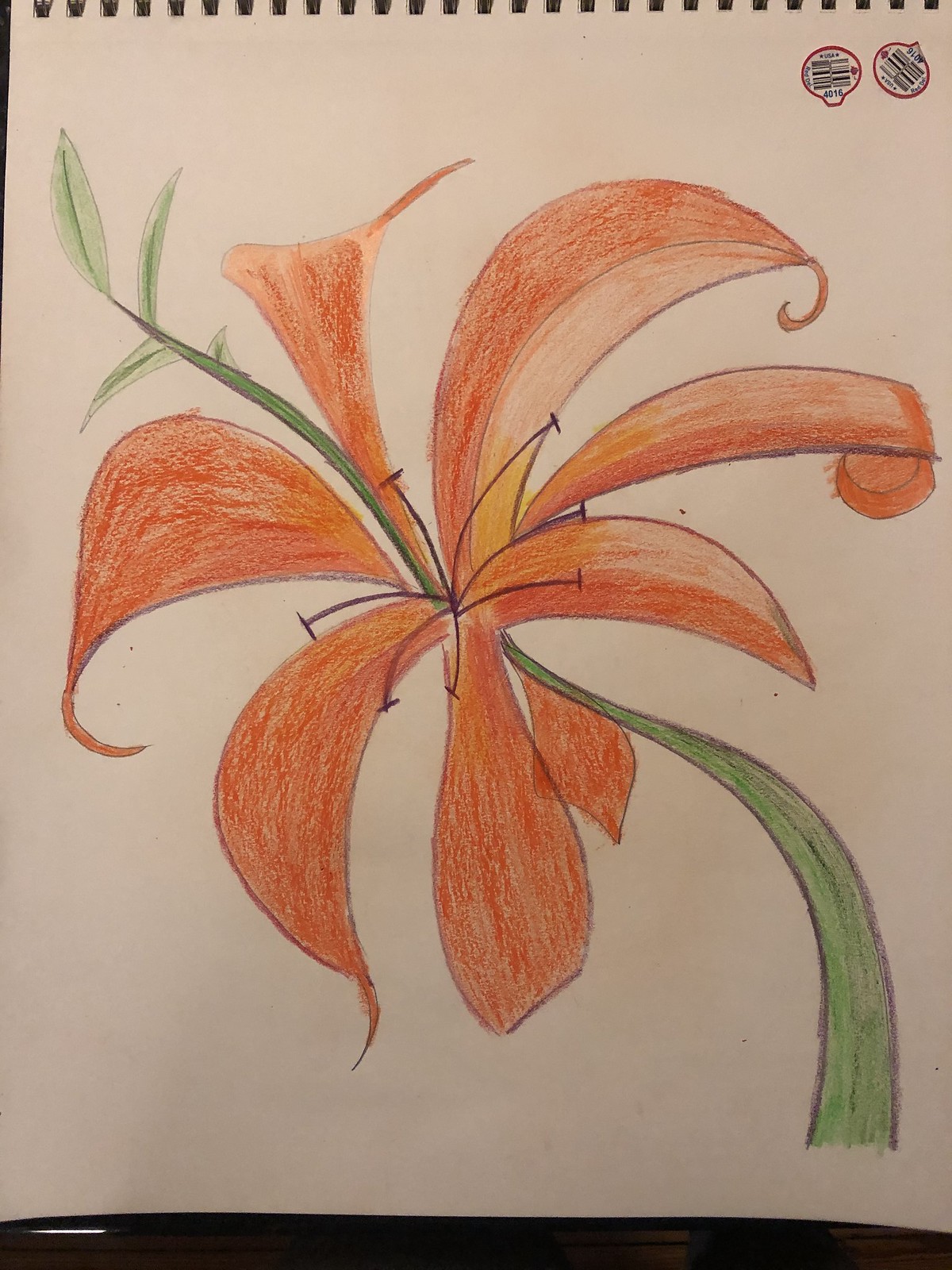The photograph showcases a hand-drawn flower meticulously illustrated with colored pencils on a blank white page within a spiral notebook. The focal point of the artwork is a large flower with striking orange petals that dominate the center of the paper. The petals curve outward from the flower's center, where delicate black stamens with tiny, pollen-less tips extend outward, adding intricate detail. The green stem of the flower winds gracefully through the petals, thickening at the base and thinning toward the top, where smaller leaves sprout. The background is starkly unadorned, highlighting the flower's vivid colors and details. In the upper right-hand corner of the page, two small stickers reminiscent of those found on grocery store fruit add an unexpected touch. These stickers feature barcodes, a red edge, and an almost speech bubble-like shape.